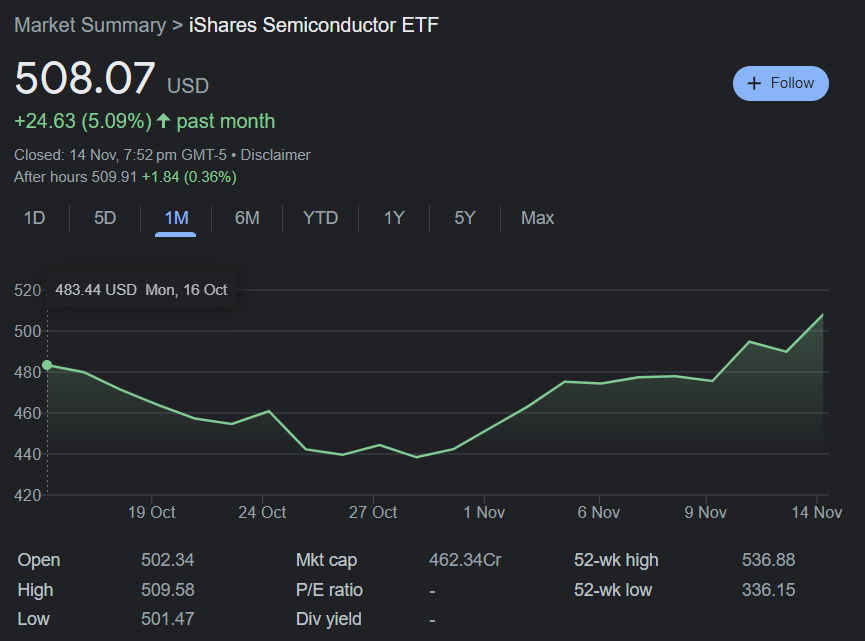The image displays a comprehensive view of the iShares Semiconductor ETF performance over time. The background features a gradient ranging from gray to black, giving a professional and analytical appearance.

In the top left corner, a section labeled 'Market Summary' stands out, followed by the ETF's full name, "iShares Semiconductor ETF," in prominent white text. Directly below, the current market price is highlighted in larger white font, showing "508.07 USD." To the right of this price, a bold blue "Follow" button is easily noticeable for quick access.

Below the listed price, a growth indicator notes a positive change, showing "+24.63" in green text with "(5.09%)" in parentheses, accompanied by an upward-pointing arrow. This data reflects the ETF's performance over the past month. Further down, in gray text, is the closing date and time: "Closed 14th November, 7:52 p.m. GMT-5," followed by a disclaimer.

Another section indicates the "After Hours" price, which is slightly higher at "509.91," with a minor increase of "+1.84" (0.36%), also noted in green.

The image includes several tabs for timeframe selection such as "1D" (1 Day), "5D" (5 Days), "1M" (1 Month) highlighted in blue, "6M" (6 Months), "YTD" (Year to Date), "1Y" (1 Year), "5Y" (5 Years), and "Max." The displayed chart below these tabs shows the ETF's price fluctuation, starting around 480, dipping slightly, and then rising again.

At the bottom, metrics regarding the ETF are provided, listing critical financial details such as "Open," "High," "Low," "Market Cap," "P/E Ratio," "Div Yield," "52 Week High," and "52 Week Low," each paired with their respective values for comprehensive analysis.

This detailed presentation allows for in-depth monitoring and analysis of the iShares Semiconductor ETF's performance and offers users clarity and actionable insights through the visual and textual data provided.